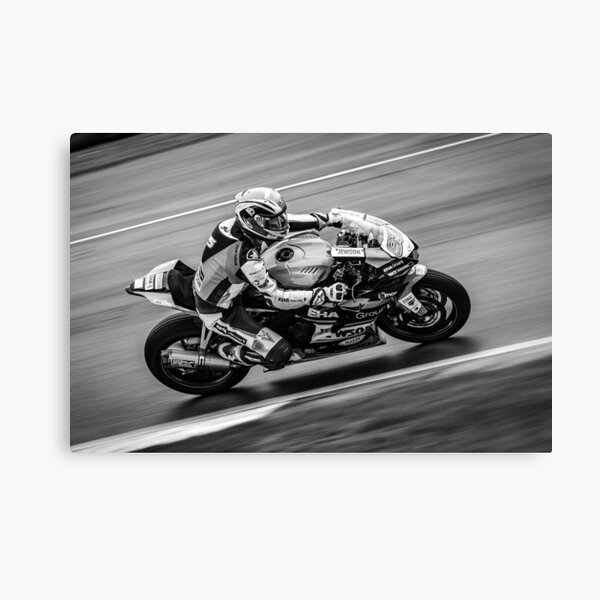This black-and-white photograph captures an exhilarating moment on a racetrack, showcasing a motorcyclist in full racing gear expertly leaning into a right-hand turn. The rider, clearly visible in great detail, wears a protective helmet, gloves, a jacket, and knee pads, embodying the focused intensity of high-speed racing. The motorcycle itself is sharp and defined against the blurred streaks of the road and surroundings, highlighting the incredible speed and motion. The contrast between the clear image of the rider and the dynamic, streaked background creates a sense of movement and adrenaline that is almost palpable.